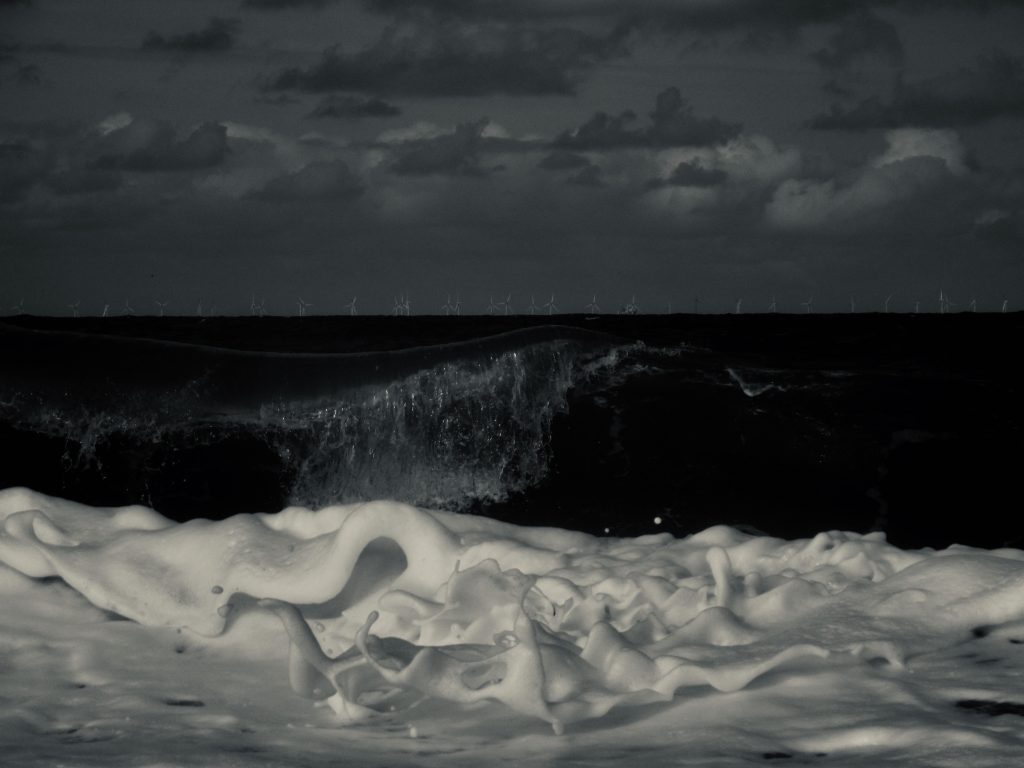This black-and-white painting captures a dramatic nocturnal seascape. The dark, almost black ocean lies in the foreground, surging with nearly milky white foam and churning waves. A significant wave, about three feet tall, is poised to crash, its crest folding over almost ten feet from a shore just outside the frame. Dense, fluffy clouds, rendered in various shades of gray, dominate the night sky, adding to the brooding atmosphere. Darker clouds interspersed with lighter, mixed ones span the gray horizon. In the distance, barely discernible objects emerge from the water, revealed to be a line of offshore wind turbines stretching across the horizon, lending an eerie yet modern touch to this moody seascape.